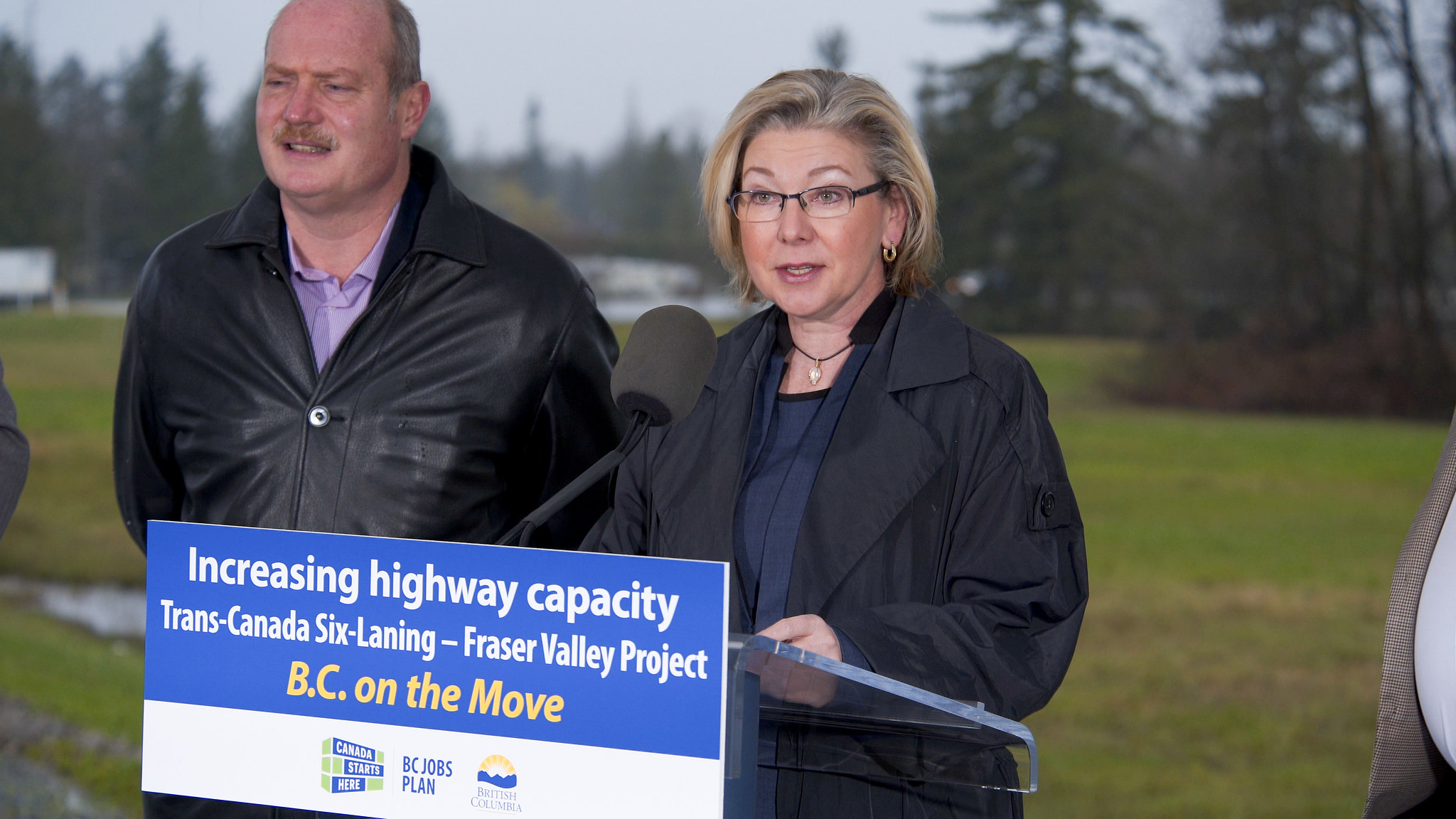In the photo, a middle-aged woman with glasses and light-colored hair stands at a clear plexiglass podium, speaking into a large black microphone. She is wearing a black jacket, possibly a raincoat, over a dark blue blouse, and has a necklace around her neck. Beside her, to the right, is a man with a receding hairline, mustache, and in a black leather jacket over a lavender shirt with an open collar. The podium displays a blue banner with the text "Increasing Highway Capacity, Trans-Canada Six-Laning Fraser Valley Project," and below in gold letters, it states "BC on the move." Additional logos for "Canada Starts Here" and "BC Jobs Plan" are also visible. The setting appears to be outdoors, indicated by the green grass, a river or body of water, and pine trees in the background, under a gray sky. The scene suggests a press conference for a highway construction project in British Columbia.